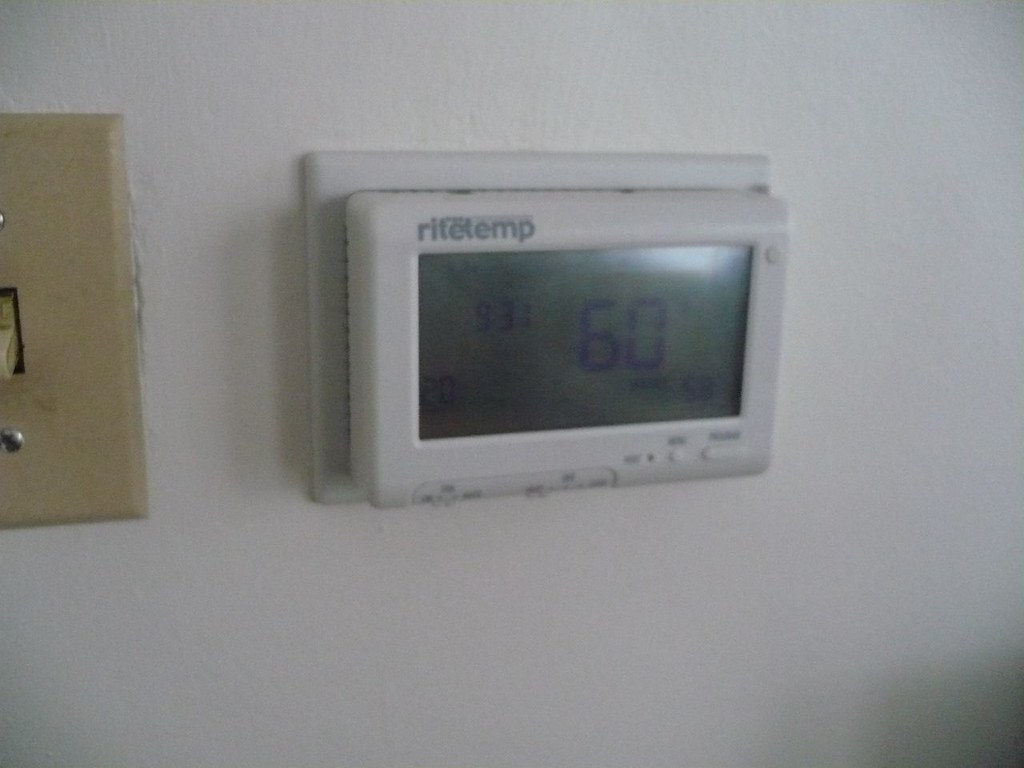A close-up photograph showcases a programmable thermostat mounted on a white wall. On the far left edge of the image, half of a light switch is visible, distinguishable by its darker tan, almost light brown color, contrasting with the white of the wall. The rectangular thermostat, oriented horizontally, features a prominent gray screen displaying "60 degrees" and "9:31" among other details. In the top left corner of the screen, the brand name "Right Temp" is clearly visible. Below the display, there are several buttons and some text, though the lower part of the thermostat is slightly blurry, making it difficult to discern the exact details. Shadows cast by the lighting create darker areas in the bottom right and top right corners of the image, adding depth to the scene.